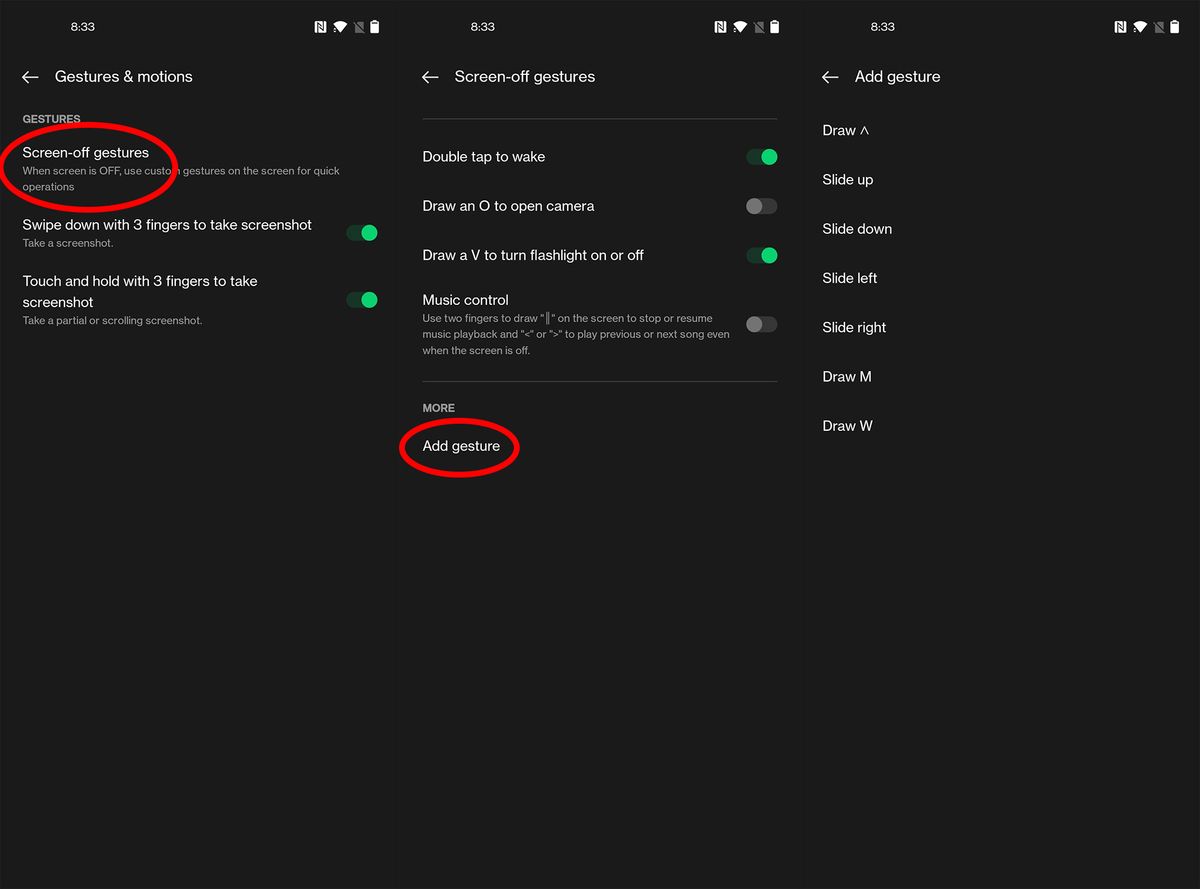The image features three Android screens against a completely black background, showcasing the configuration and options available for gestures and motions. The first screen, outlined in white font, headlines "Gestures and Motions" and lists options under "Screen Off Gestures." Here, two functions are specified: "Swipe down with three fingers to take a screenshot" and "Touch and hold with three fingers to take a screenshot." This screen highlights the "Screen Off Gestures" section with a red circle.

Moving to the second screen, titled "Screen Off Gestures," additional gesture options are displayed. These include: "Double-click to wake" (turned on), "Draw an O to open camera" (turned off), "Draw a V to turn flashlight on or off" (turned on), and "Music control" (turned off). At the bottom, there are "More" and "Add Gesture" options, with the "Add Gesture" option circled in red.

The third and final screen, labeled "Add Gesture," offers a variety of gesture options such as "Draw an up arrow," "Slide up," "Slide down," "Slide left," "Slide right," "Draw M," and "Draw W." Interestingly, the arrangement of these screens appears to be in reverse order, suggesting a step-by-step navigation through the gesture settings.